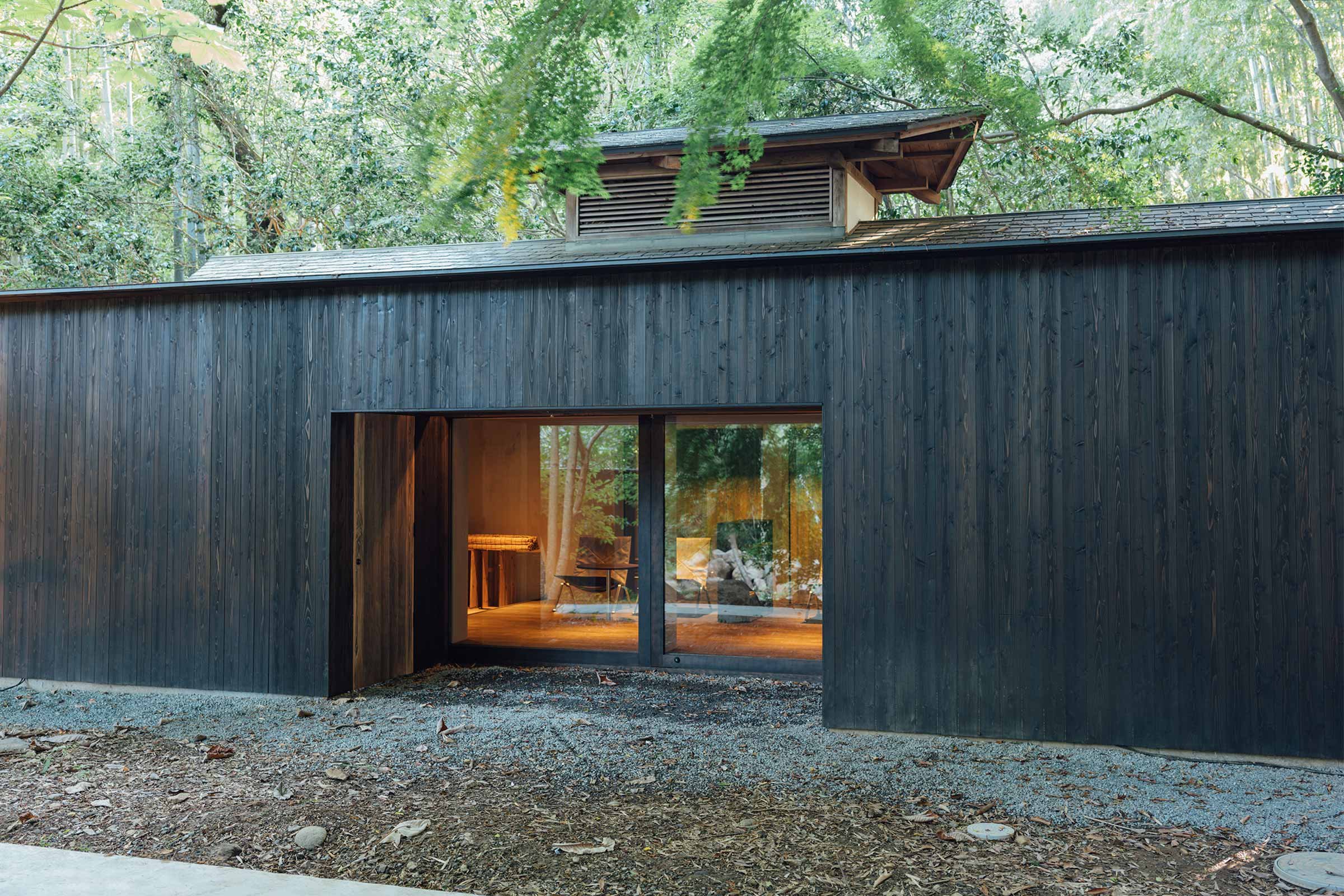In this detailed outdoor image, we see a rustic, rectangular building clad in dark brown vertical wooden planks, with a low-slope shingle roof. The building’s design includes a notable vented protrusion on the roof, contrasting with the main structure. Dominating the front are two large, transparent windows that offer a glimpse into the interior, revealing chairs and a hardwood floor, and even providing a view straight through to trees in the background. The structure sits amidst a dirt foreground speckled with leaves, alongside a sidewalk visible in the lower left corner. Surrounding the building are tall, lush deciduous trees, their branches overhanging and appearing to nearly touch the roof, enhancing the natural and somewhat secluded ambiance of the scene.